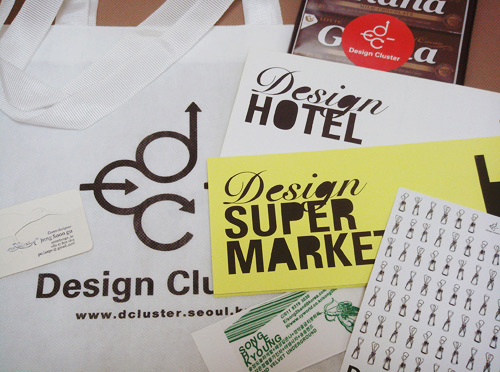The photograph depicts a cluttered table, strewn with various promotional materials and freebie items. Dominating the left side is a white reusable tote bag with straps folded down. The bag features a logo consisting of a "D" with an upward arrow, a "C" with a rightward arrow, and another "C" with a circular arrow, accompanied by the text "Design Club" and the partially visible URL "www.decluster.sol." Resting atop the bag is a business card obscuring some details. Scattered across the table are several more business-type cards and brochures. Notably, a yellow card with black text reading "Design Supermarket" overlaps a white card inscribed with "Design Hotel." In addition, a sheet of stickers or stamps is visible in the upper-right corner, adding to the assortment of scattered advertising materials.